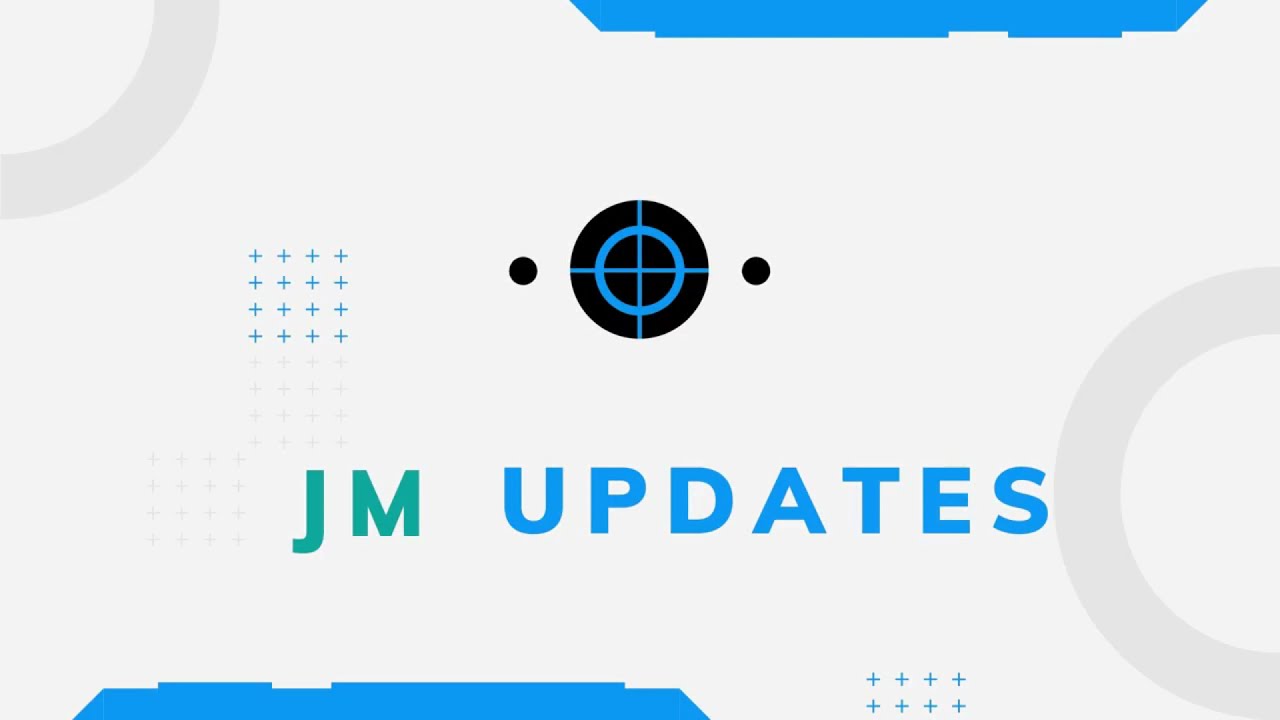This digital image features a graphical design set against a light off-white backdrop with distinct patterns and text elements. Dominating the center is a circular pattern resembling a black and blue bullseye. Flanking this bullseye on either side are two small black dots. Surrounding the central element, there are various grids of blue plus signs: a 4x4 grid situated above the text area and a 4x2 grid below it. Toward the upper left corner and the lower right corner, there are darker gray arch-like semi-circles. Along the top edge and the bottom left edge of the image are thin blue parallelograms with intricate designs. At the bottom of the image, in green and blue capital letters, the text reads "JM UPDATES," with "JM" in green and "UPDATES" in blue.